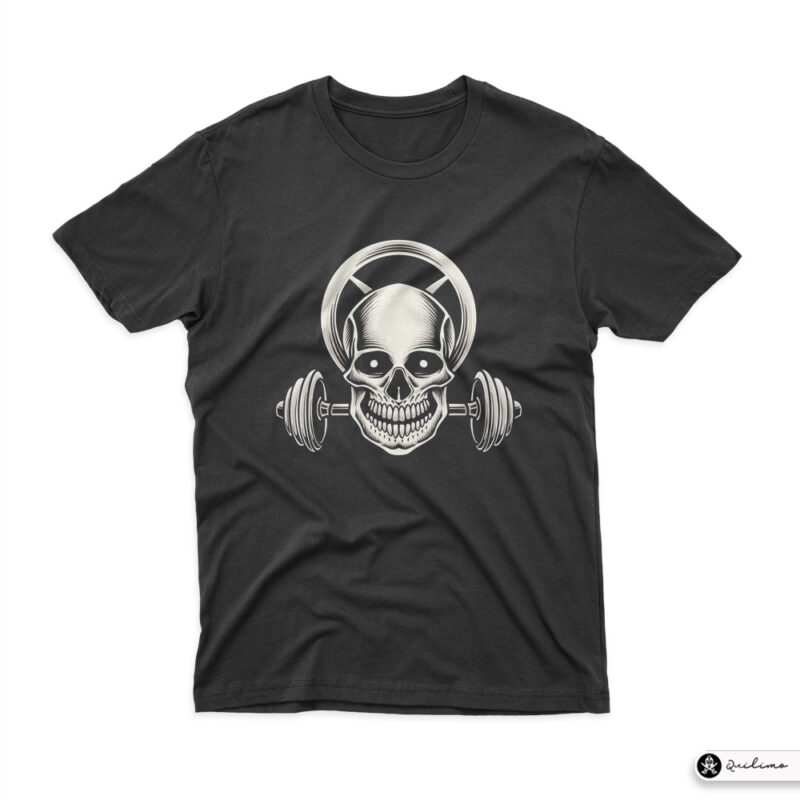The image portrays a dark charcoal black t-shirt, photographed from above against a white background in a black-and-white portrait orientation. The t-shirt features a graphic that dominates the center of the chest area. This graphic presents a large, menacing skull facing the viewer with a broad, tooth-filled smile. The skull has dark eye sockets each containing a small white dot, giving it an eerie and haunting expression. Behind the skull, there is a radial wheel-like structure that resembles either a crown or a halo, from which two spikes protrude upwards on each side.

The skull's design is further embellished with a barbell that runs horizontally behind its teeth, each end fitted with sets of weights. On each side of the barbell, there are three circular weights. The t-shirt itself is slightly wrinkled, with noticeable creases running from the top right shoulder towards the center of the chest, from the neck down halfway to the left, and several more near the elbows and the bottom hem.

Detailing the finishing touch, in the bottom right corner of the t-shirt, there is a small white tag with an intricate, unreadable black cursive logo, and to the left of the tag is another small skull symbol. The overall style of the photograph is highly detailed, leaning towards a realistic and representational approach typical of professional product photography.